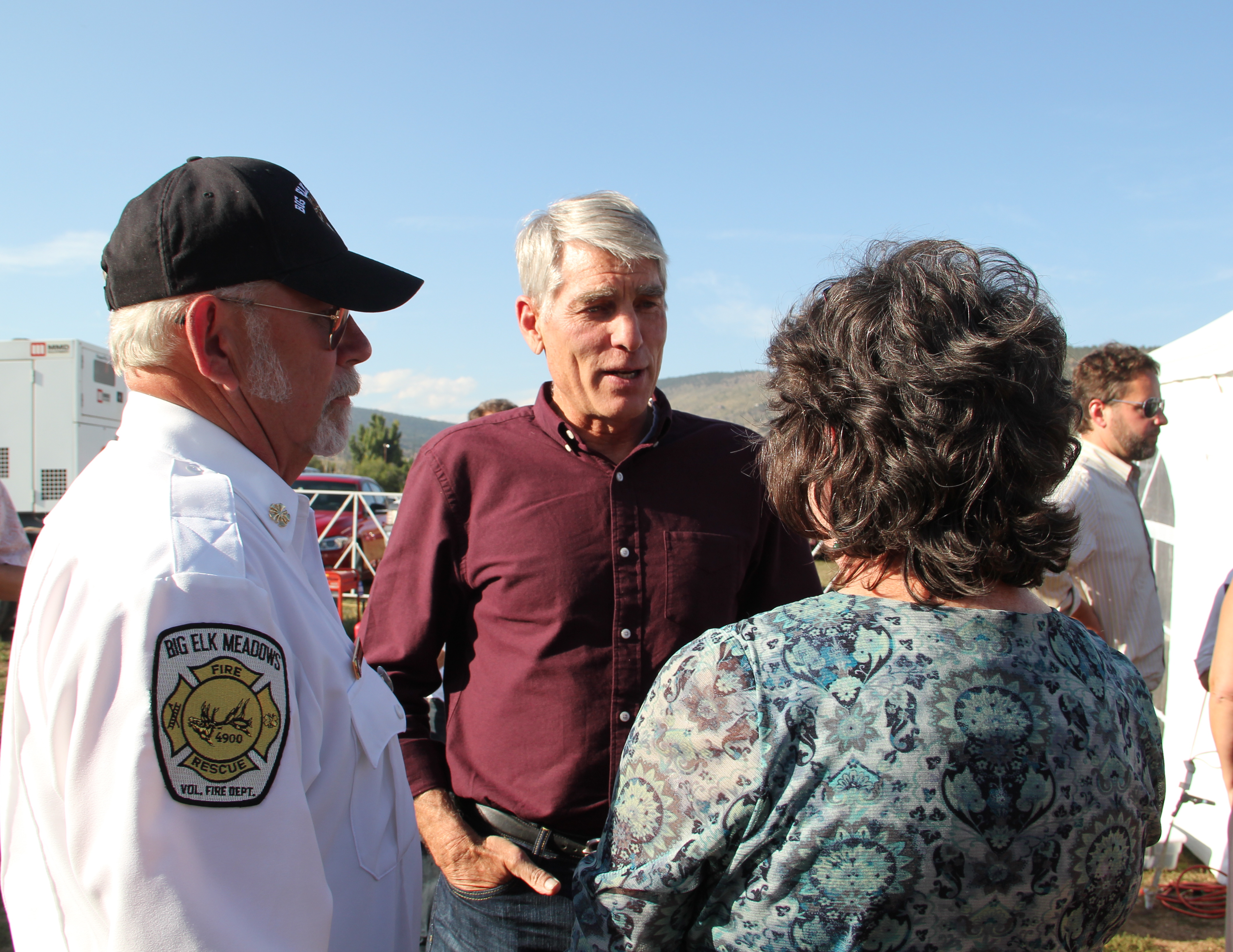In the image, an older gentleman wearing a maroon button-down shirt with blue jeans stands with his right hand in his pocket, conversing with a woman whose back is visible to us. She sports a shoulder-length, dark hair, cut shorter on the sides, and is dressed in a blue paisley-patterned shirt that contains lighter colors. To the right of the woman, a man in a white shirt and sunglasses stands next to a white tent. Nearby, a Big Elk Meadows Fire Rescue volunteer, identifiable by his white shirt, black baseball cap, gold collar tack, and a patch on his right shoulder that includes the words "Big Elk Meadows Fire Rescue," listens attentively.